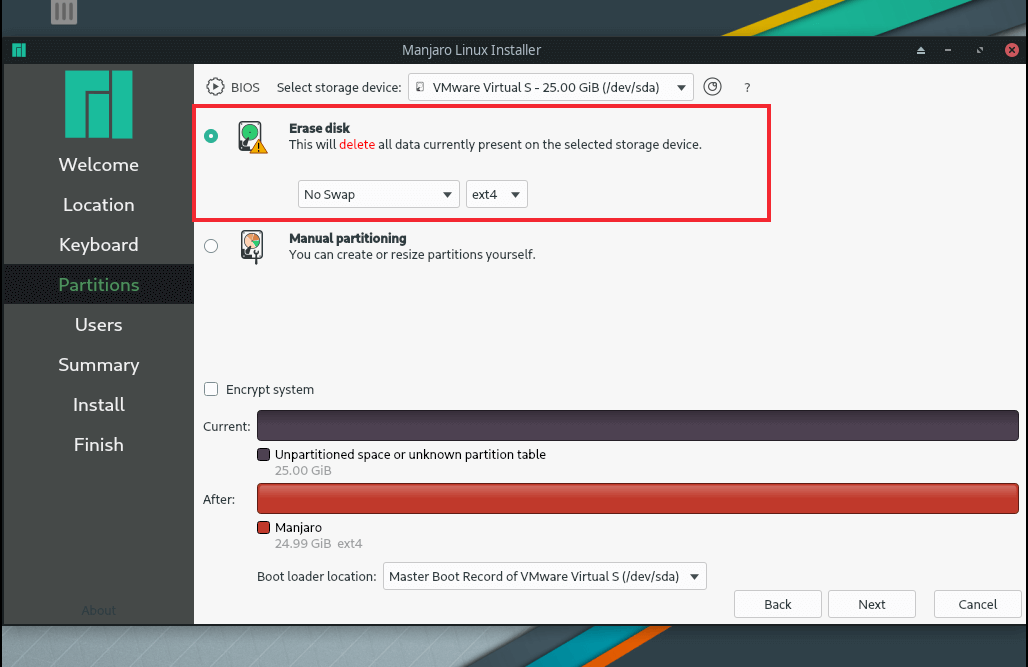This image is a screenshot of the Manjaro Linux Installer web page. At the very top, the title "Manjaro Linux Installer" is prominently displayed. On the left-hand side, there is a vertical column featuring a teal box designed to resemble interlocking puzzle pieces. A smaller, identical teal puzzle piece is located in the upper-left corner of this column.

Below the teal box, a list of installation steps is outlined in white text on a gray background. The steps read: "Welcome," "Location," "Keyboard," "Partitions," "Users," "Summary," "Install," and "Finish." The "Partitions" step is selected, highlighted with a black background, and the word "Partitions" itself is displayed in green.

In the main content area, a red rectangle prominently highlights the "Erase Disk" option. Below this, you can see options for system encryption, labeled "Encrypt System," with sections for "Current" and "After." The "Current" section features a long black line, while the "After" section is indicated by a red line.

Lastly, there is a key that reads "Manjaro" in the bottom section of the screenshot.